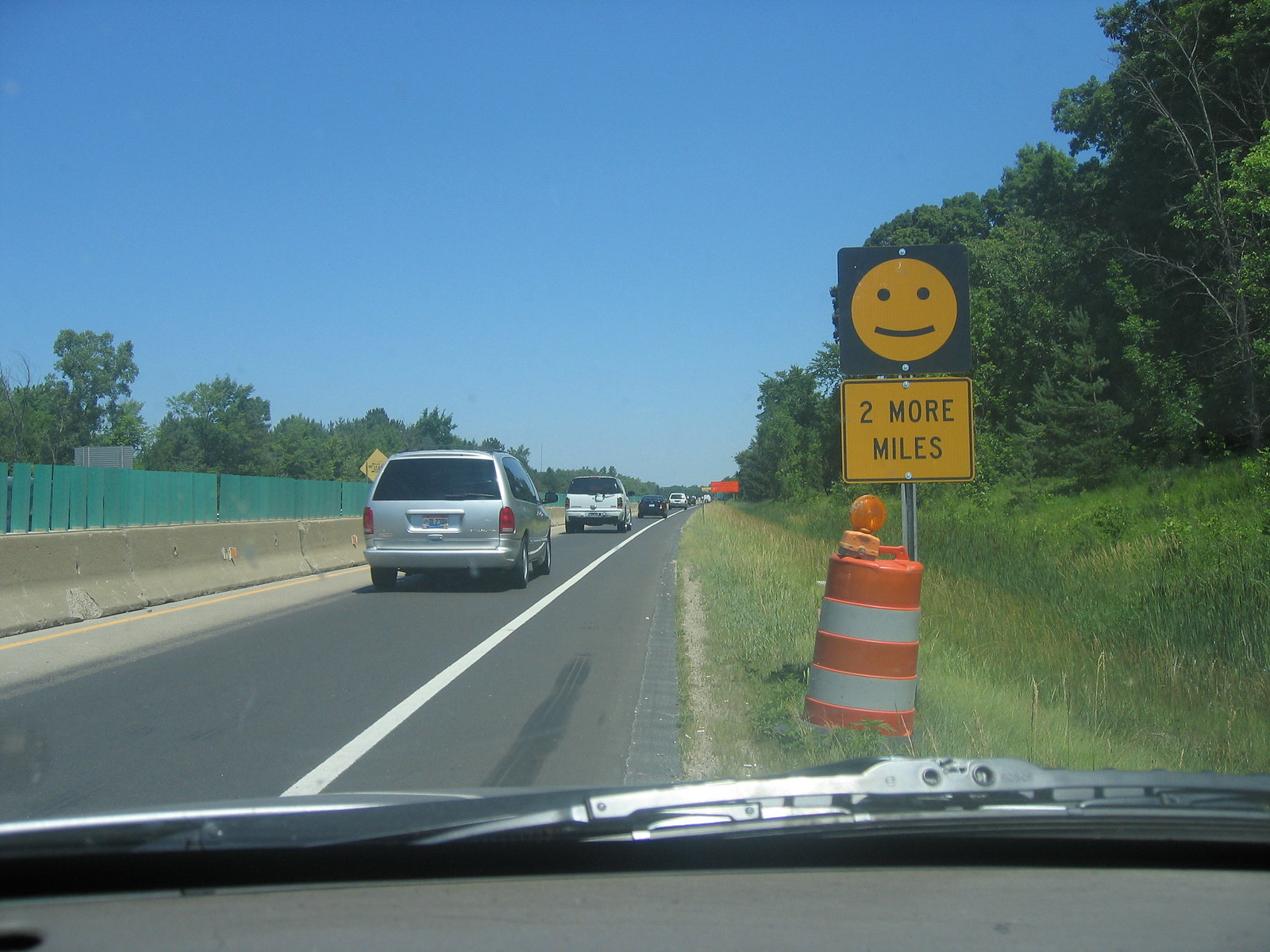A real-life image captured from inside a car parked in the emergency shoulder lane on the right side of a single-lane road. In the foreground, a plastic orange bin with orange and white stripes sits prominently, adorned with a flashing yellow construction light. Behind it, a metal pole supports two signs: the bottom one is a yellow square with a black border displaying the text "TWO MORE MILES" in all capital letters, and the top sign features a yellow smiley face on a black background, reminiscent of an emoji.

The metal post is situated in a grassy area that seamlessly merges into the asphalt road without a distinct border, creating a ravine-like dip before rising into a dense, forested area. The road itself is busy, with about four or more cars visible in the distance. The closest vehicle in the actual lane is a silver van, followed by a white SUV, a black sedan, and another distant white car.

To the left of the road, a cement barricade topped with a green fence extends along the side, with the upper canopy of trees visible behind it. The sky above is a clear blue, void of clouds, indicating a bright, sunny day.